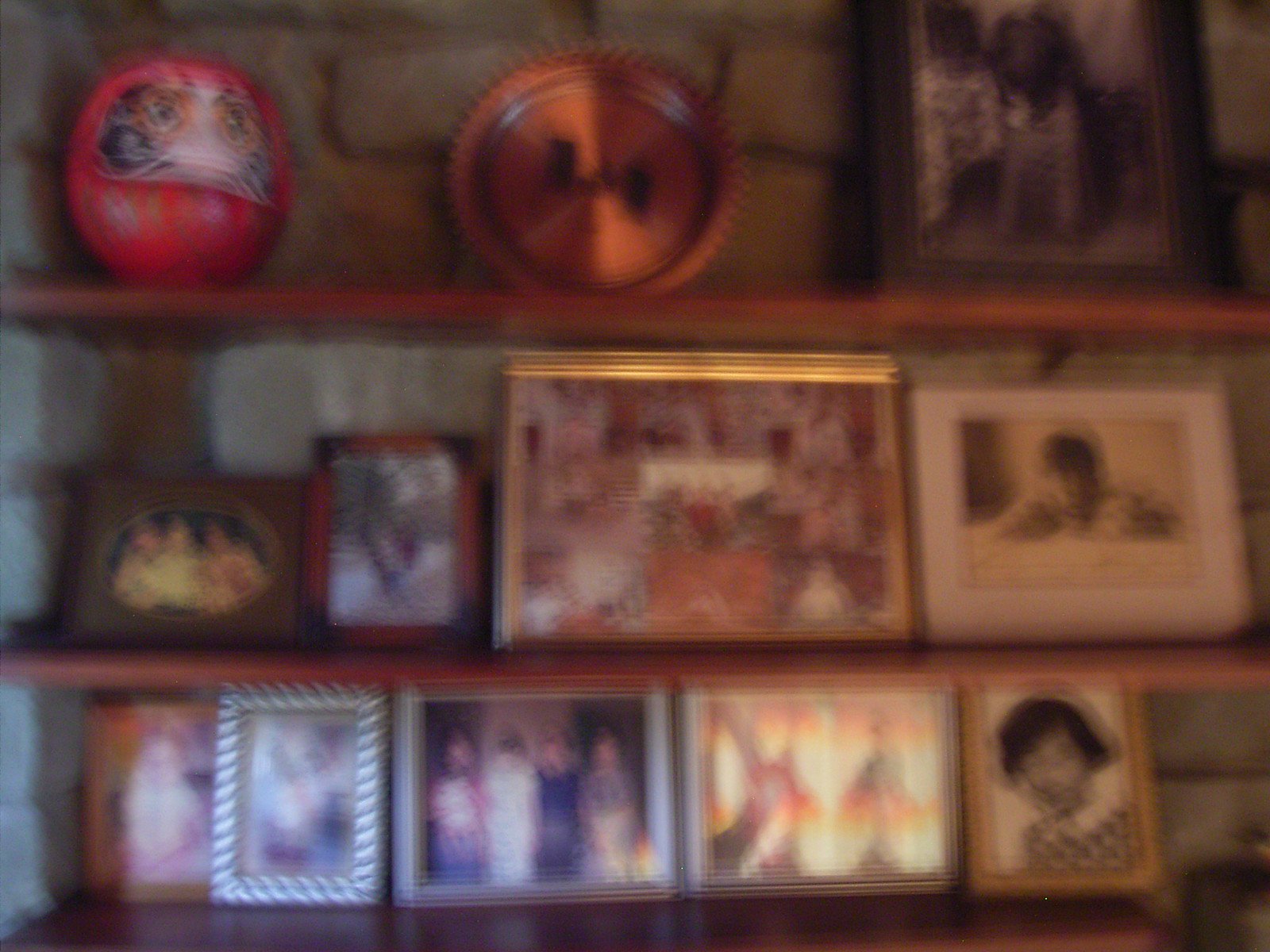In this image, a slightly fuzzy photograph captures a shelf adorned with a collection of ten framed pictures. The frames are arranged with five on the bottom row, four in the middle, and one perched on the top. To the right of the solitary top frame, a brass plate, perhaps a decorative item, is positioned centrally. On the far left-hand corner of the shelf, a pink toy with prominent green eyes and an orange and white face, resembling a cat, adds a whimsical touch to the display. Despite the blurriness of the image, the organized arrangement and the distinctive details of the toy are discernible.